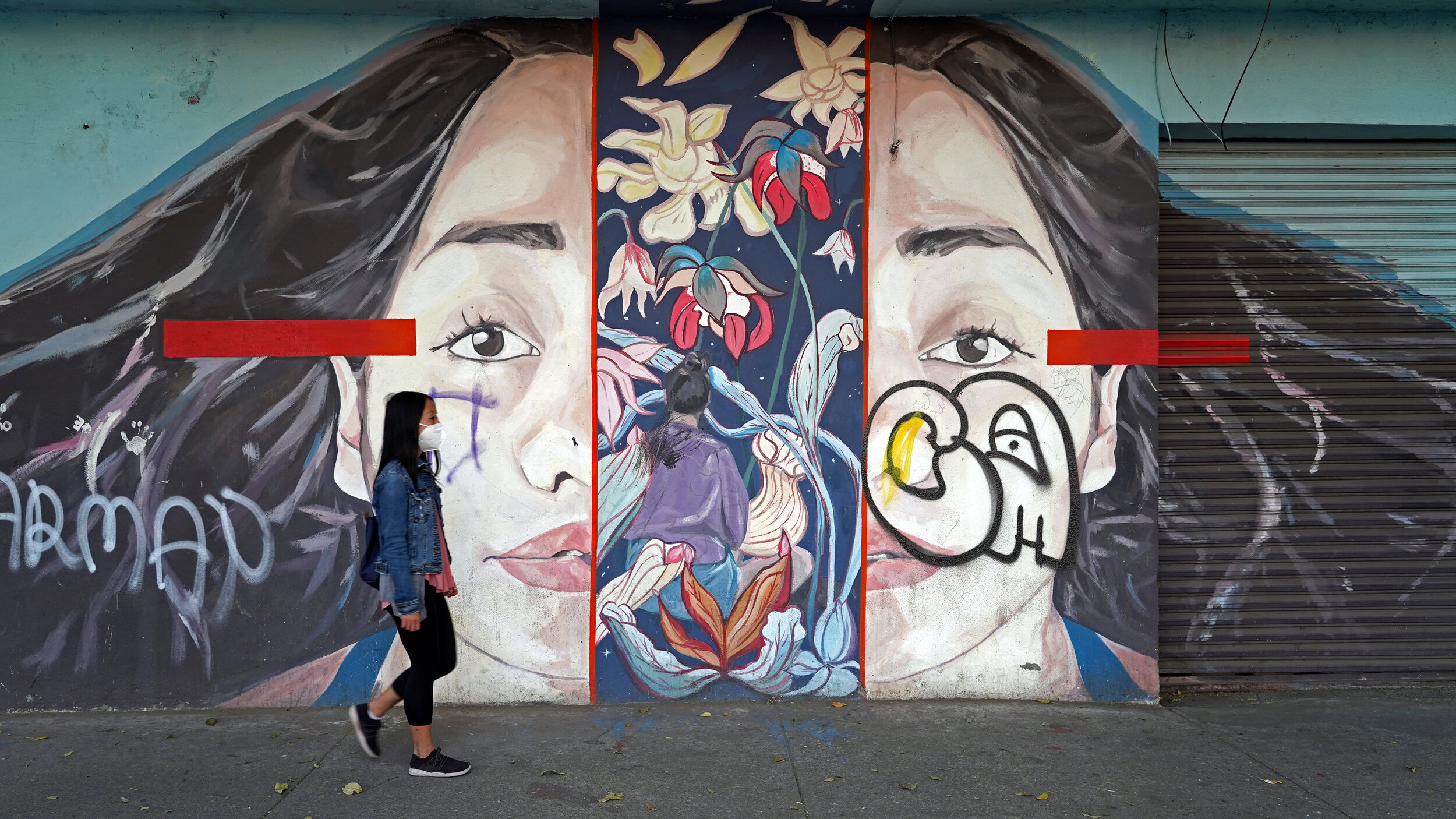This vibrant color photograph captures a striking mural painted on a wall, depicting the face of a woman with long, dark hair. The artwork is intricately designed, with her face bisected vertically to reveal a whimsical panel showing tall, blooming flowers. Within this floral expanse, a figure sits with their back to the viewer, gazing contemplatively at the blossoms. The mural is adorned with graffiti; on the left side, someone has spray-painted "ARMA" in loopy white letters accompanied by a white handprint above it. On the right side, the letters "C" and "A" are prominently spray-painted, adding to the urban aesthetic. Walking in front of the mural is an Asian woman with long, dark hair, clad in a denim jacket layered over a pink top, black leggings, and black sneakers. She is also wearing a white face mask, blending contemporary street style with pandemic-era vigilance.